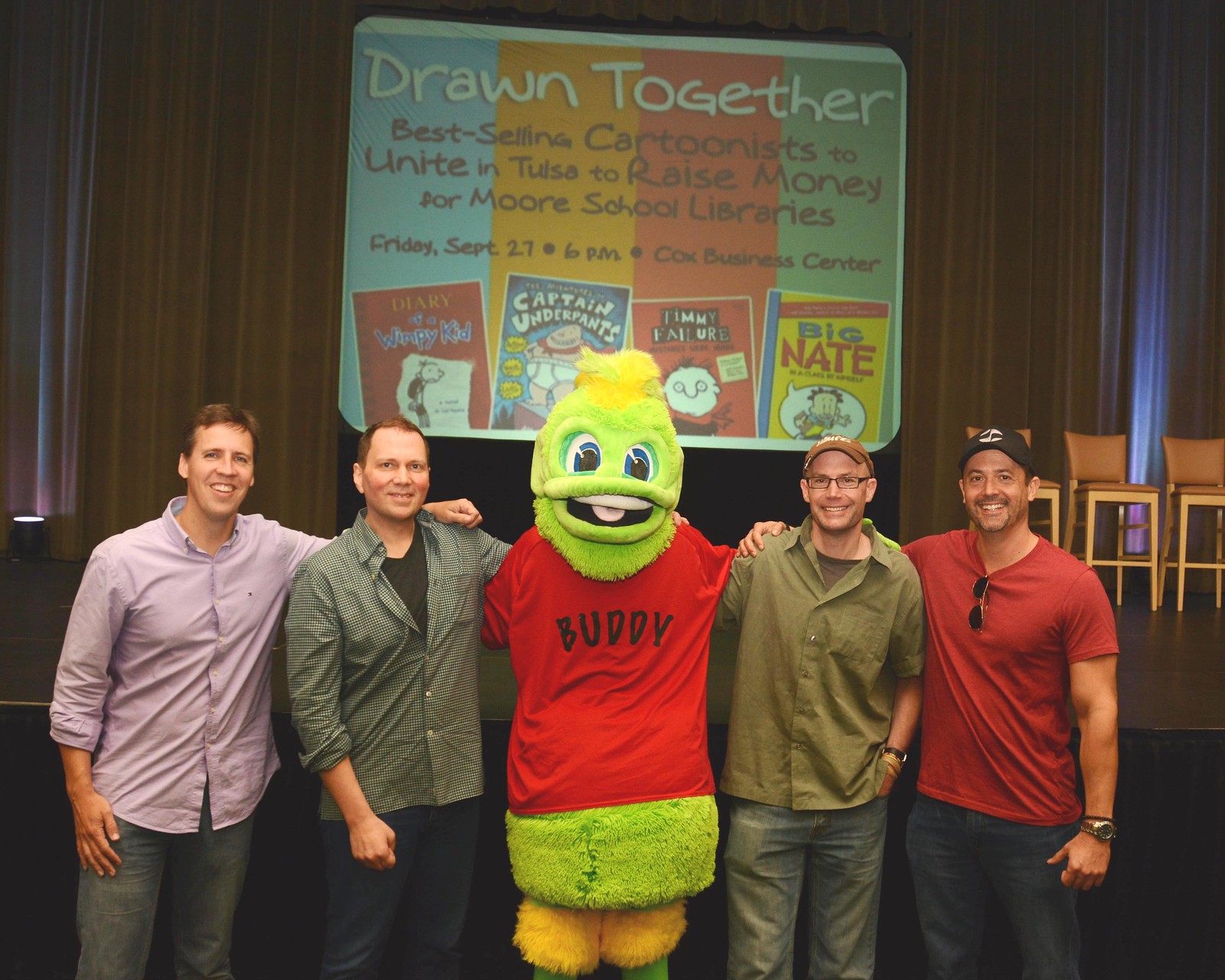The image depicts four middle-aged men standing around a large, neon green duck mascot named Buddy, who is dressed in a red t-shirt with "Buddy" written in black on it, a yellow bottom, and green-and-yellow boots. From left to right, the men are: one in a lavender shirt and jeans, another in a greenish button-down shirt with a black undershirt and jeans, the third in a green shirt with a brown undershirt, glasses, a brown baseball cap, and jeans, and the fourth in a red shirt with a blue baseball cap, sunglasses dangling from the shirt, and jeans. They are posing in front of a stage with a black backdrop. Behind them, a large banner reads: "Drawn Together: Best Selling Cartoonists to Unite in Tulsa to Raise Money for More School Libraries." The banner features vibrant colors such as blue, yellow, red, and green, and includes images of cartoons created by the artists. Additionally, there is a projector screen listing the event details, which specifies the date as Friday, September 27, 6 p.m. In the lower right corner of the image, some brown chairs are visible. The setting is clearly an interior space, likely a theater, illuminated by artificial lighting.